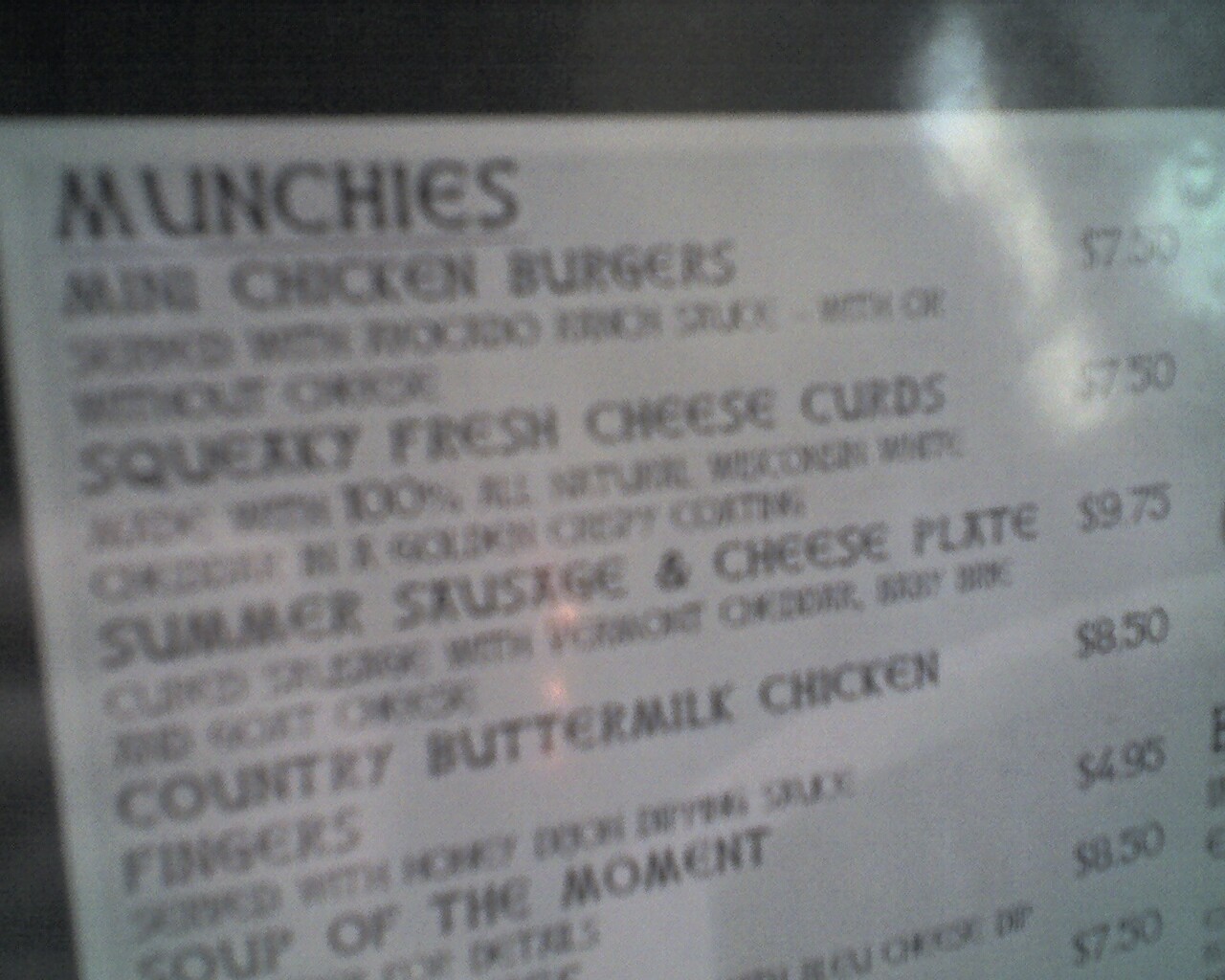This color photograph captures a slightly out-of-focus menu sign set against a dark backdrop. The white sign features black text at the top proclaiming "Munchies." Despite the blurriness, the menu items are still legible. 

1. **Chicken Burger** - Priced at $7.50, includes a list of ingredients.
2. **Squeaky Fresh Cheese Curds** - Costing $7.50.
3. **Summer Sausage and Cheese Plate** - Available for $9.75.
4. **Country Buttermilk Chicken Fingers** - Priced at $8.50.
5. **Soup of the Moment** - Offered at $4.95.

There are additional items with prices listed at $8.50 and $7.50, but their names are cut off and not visible in the photograph. The dim lighting in the background accentuates the menu sign's presence, highlighting its offerings for passersby despite the slight blurriness of the text.